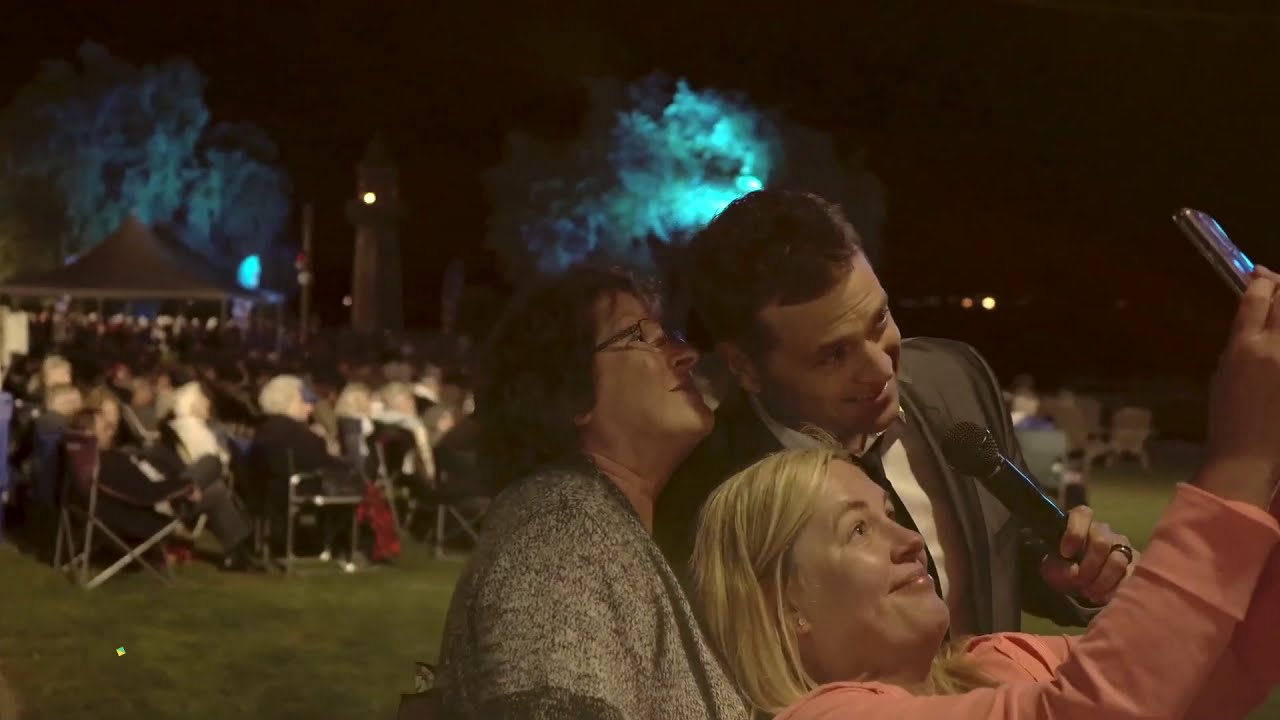In this detailed photograph taken outdoors at night during a large event, we see a dynamic trio taking a selfie. The primary focus is a blonde woman with straight hair, wearing a tangerine-colored long-sleeved shirt, leaning back and holding a phone above her to capture the moment. Flanking her are two others: an older woman with short brown hair and glasses, dressed in a gray and black sweater, and a gentleman with short brown hair, attired in a gray suit, white shirt, and loosened black tie, holding a microphone in his left hand, indicating he might be a reporter or some notable figure. They appear cheerful and are closely huddled to fit into the selfie. Behind them, a festive scene unfolds with numerous older attendees seated on the grassy lawn, illuminated by lights in the trees and possibly gearing up for a concert or fireworks. In the distance, one can spot a blue glow and silhouetted mountains, enhancing the ambiance of the event.